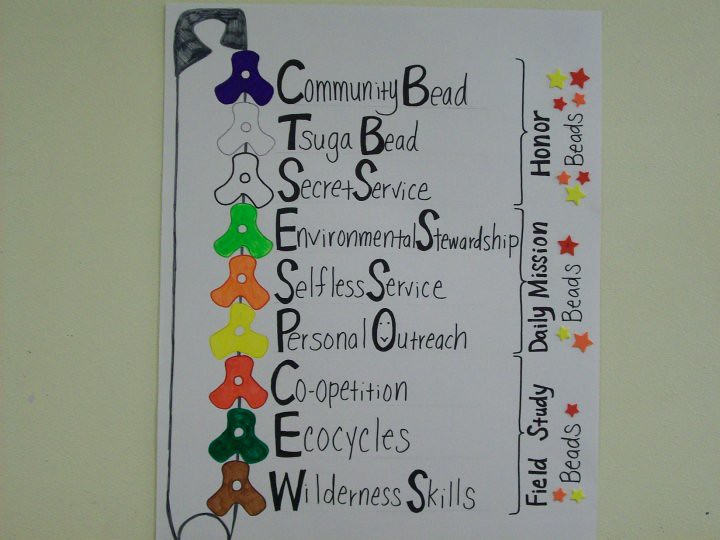The image depicts a hand-drawn poster hanging on a white wall. Centrally placed on the poster, a list of categories is written in a vertical arrangement, with the first letter of each word capitalized twice as large as the rest. The categories include: Community Bead, Sugaga Bead, Secret Service, Environmental Stewardship, Selfless Service, Personal Outreach, Co-opetition, Eco-cycles, and Wilderness Skills.

On the right side of the poster, heading from bottom to top instead of left to right, are the labels: Field Study Beads, Daily Mission Beads, and Honor Beads. Each of these categories is in parentheses, grouping the previously mentioned categories into sections.

The left-hand side of the poster features colorful, triangular flower puzzle pieces in shades of purple, white, green, orange, and yellow, forming an intricate pattern that appears stacked and overlapping. Below this floral design, there is a geometric tube-like pattern. Scattered throughout the different bead categories on the right are small yellow and orange stars, adding extra color and visual interest to the display.

This poster seems to be intended for an educational or work setting, given its mix of structured text and decorative elements.